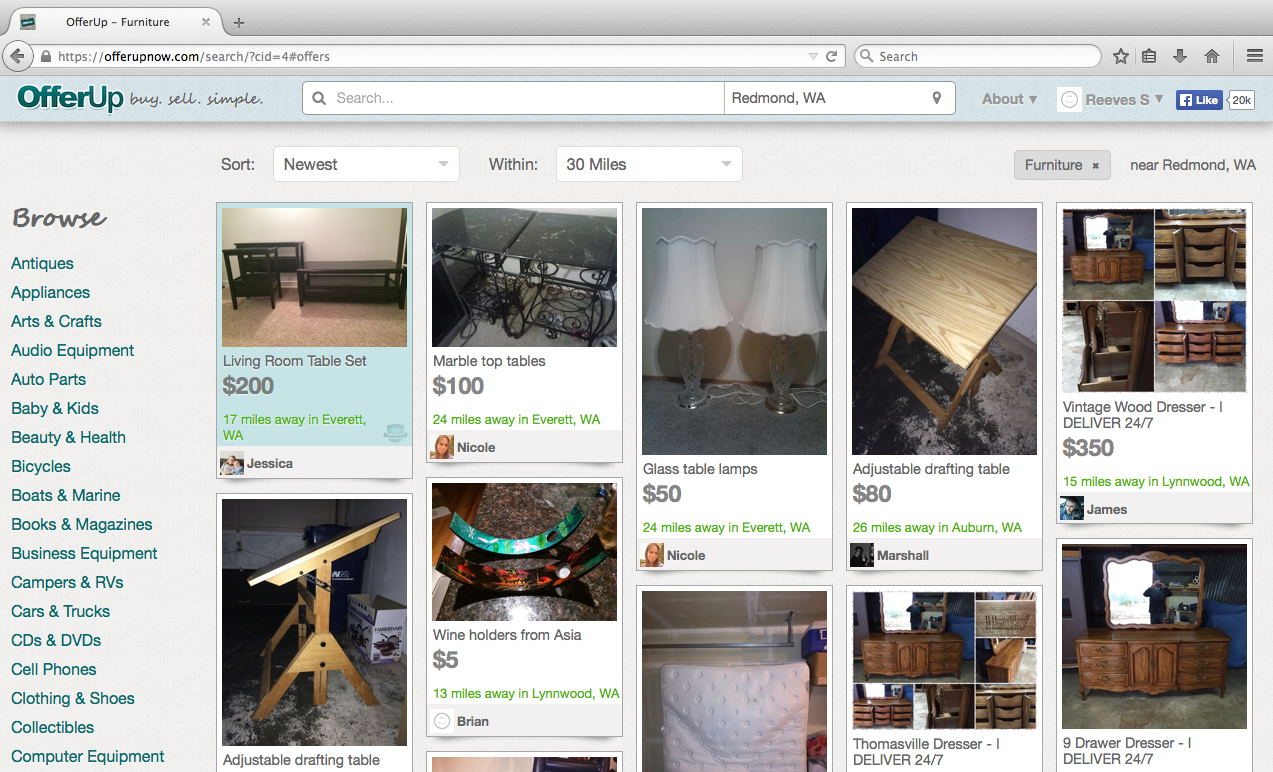A screenshot of a web page from an OfferUp search for furniture is shown. The top banner is gray, displaying a tab labeled "OfferUp-Furniture" with a capital "O" and "U". An avatar for OfferUp is visible on the left. Below, a gray back arrow is adjacent to a gray lock icon in the address bar, which reads "https://offerupnow.com/search/?CID=44". To the right are a refresh button, a search bar with a magnifying glass icon, and icons for a star, a clipboard, a down arrow, a house silhouette, and three horizontal lines.

Below the gray banner, a light blue banner features "OfferUp" in aqua turquoise with "Buy. Sell. Simple." in gray cursive. Another search bar reads "Redmond, Washington" with a location symbol. Further descriptions include an "About" section with a down arrow, a white square with a smiley face captioned "Reeves S.", and social media icons.

The page allows sorting with "Newest" selected and within "30 miles" of Redmond, Washington, under the category "Furniture." The "Browse" section in cursive features categories such as "Antiques," "Appliances," "Arts and Crafts," "Audio Equipment," "Auto Parts," "Baby and Kids," "Beauty and Health," "Bicycles," "Boats and Marine," "Books and Magazines," "Business Equipment," "Campers and RVs," "Cars and Trucks," "CDs," "DVDs," "Cell Phones," "Clothing and Shoes," "Collectible," and "Computer Equipment."

A grid of images displays:

1. **Living Room Table Set** - $200, located 17 miles from Everett, WA, highlighted in green.
2. **Marble Top Tables** - $100, located 24 miles from Everett, WA, sold by Nicole (avatar displayed).
3. **Black Equipment with Cables** - $100, located 24 miles from Everett, WA, sold by Nicole (avatar displayed).
4. **Glass Table Lamps** - $50, located 24 miles from Everett, WA, sold by Nicole (avatar displayed).
5. **Oak Wood Coffee Table** - Adjustable drafting table for $80, located 29 miles from Auburn, WA, sold by Marshall (avatar partially visible).

Other listings include:

- **Vintage Wood Dresser** - $24-$750, located 50 miles from Linwood, WA.
- **Adjustable Drafting Table** - Shows a brown wooden table frame with a white box in a soiled garage.
- **Wine Holders** - Describe brown items with neon green and red rings.
- **Leather Bound Books Collection** - Thomasville dresser with 24-7 delivery.
- **Nine-Drawer Dresser with Mirror** - Delivered 24-7, featuring a dog walking on it.